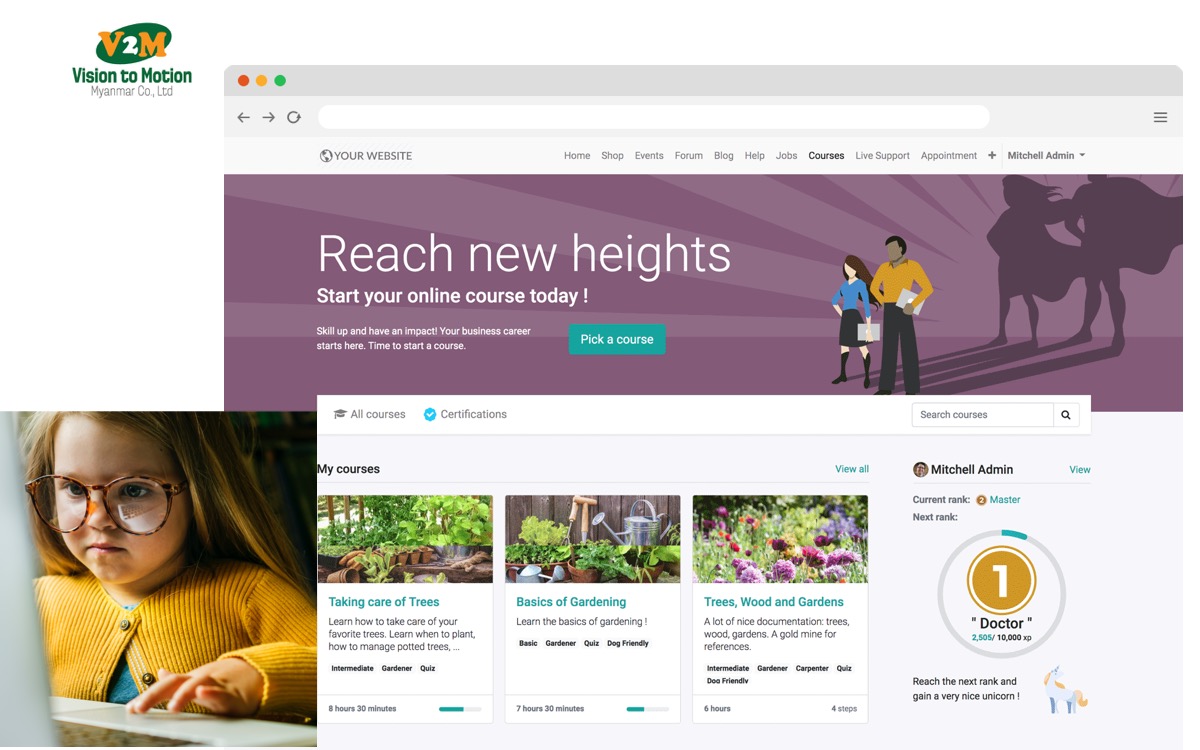In the top left corner of the image, there is a slightly slanted dark green oval with its top edge angled towards the upper right. Inside the oval, there is a stylized, bubbly orange letter 'V' followed by a similarly styled '2' in the center, and finally, an orange letter 'M'. Below this logo, "Vision to Motion" is written in green font. Underneath this tagline, the words “Myanmar, Colorado, LTD” are written in gray.

To the right side of the image, a web page is displayed on a device, possibly a MacBook or an iPad, identifiable by the characteristic light gray header with rounded corners and the traditional red, yellow, and green dots at the top left of the screen. The webpage’s header reads "Your Website," indicating it might be a template. On the right side of the page, there is a menu in gray text displaying options: Home, Shop, Events, Forum, Blog, Help, Jobs, Courses. The "Courses" option is highlighted in bold black. Under this menu, there is text that reads "Live Support Appointment" followed by a bold plus sign, then a light gray divider line. Below the divider, it says "Mitchell Admin" in bold gray font, accompanied by a dropdown arrow.

The background of the image is a dark purple, with a light purple beam emanating outward. Centered within this background is a man with his hands on his hips, holding a book. He is dressed in a yellowish-orange shirt. To his right stands a woman wearing a blue shirt and a black skirt, also holding a book. Their reflections and shadows are visible to the right of them. On the left side of the image, the text "Reach New Heights" is written in bold white lettering. Below this, in smaller but bold white text, it says "Start Your Online Course Today!"